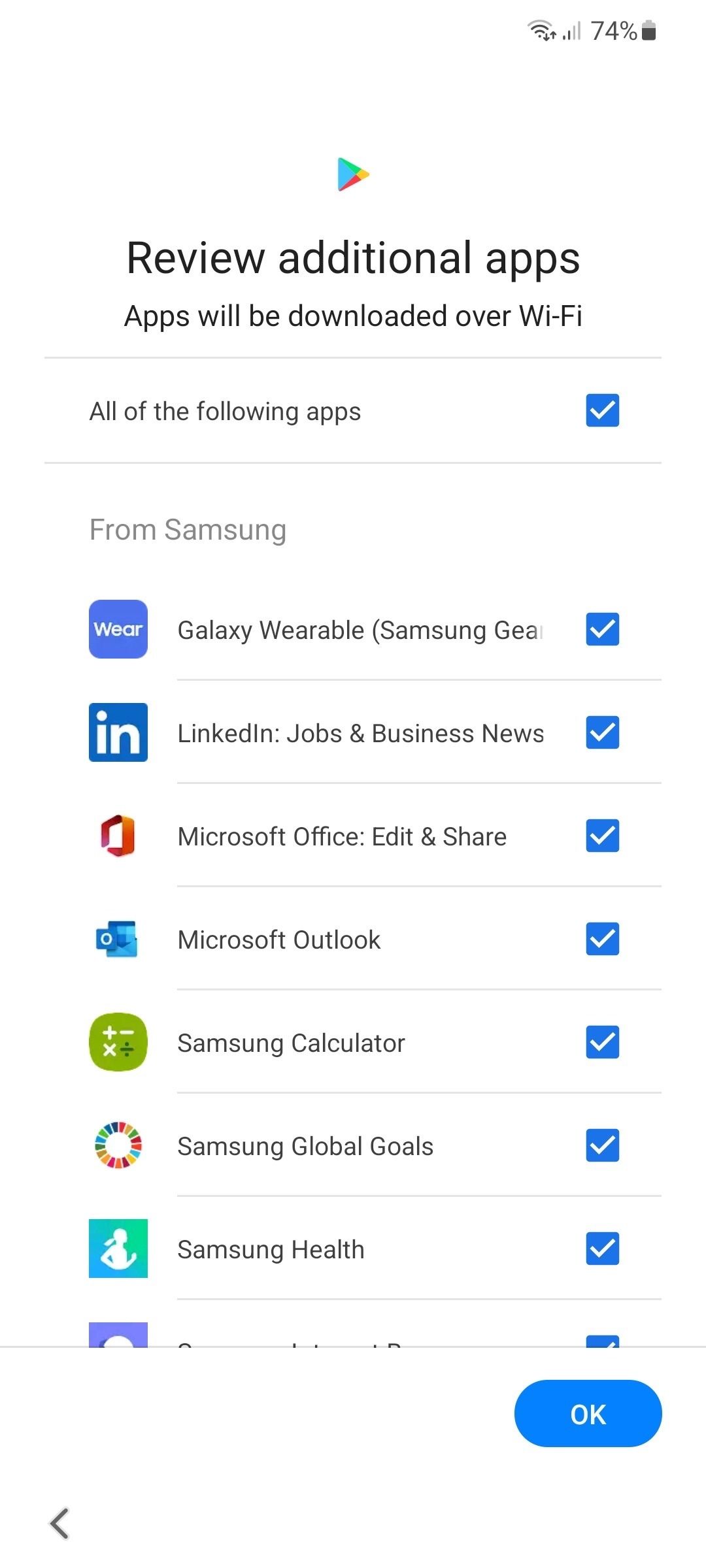The image is a detailed screenshot from a smartphone displaying a list of additional apps available for download. At the top, there is a Google icon followed by the Play Store icon, characterized by a right-facing triangle composed of red, yellow, blue, and green shapes. The heading reads "Review Additional Apps," with a subtitle indicating that "Apps Will Be Downloaded Over Wi-Fi."

Below this heading, a checklist appears showcasing various apps that can be selected for download. This list is titled with another subtitle, "From Samsung." There are approximately eight Samsung-related apps listed, each accompanied by its icon on the left. The listed apps include:

1. **Galaxy Wearable (Samsung Gear)**
2. **LinkedIn (Jobs and Business News)**
3. **Microsoft Office (Edit and Share)**
4. **Microsoft Outlook**
5. **Samsung Calculator**
6. **Samsung Global Goals**
7. **Samsung Health**
8. **An app with a recognizable logo but unnamed in the text**

All the apps in this list are currently checked, indicating they are selected for download. At the bottom right of the screen, an "OK" button is present, likely to confirm the selection and proceed with the download.